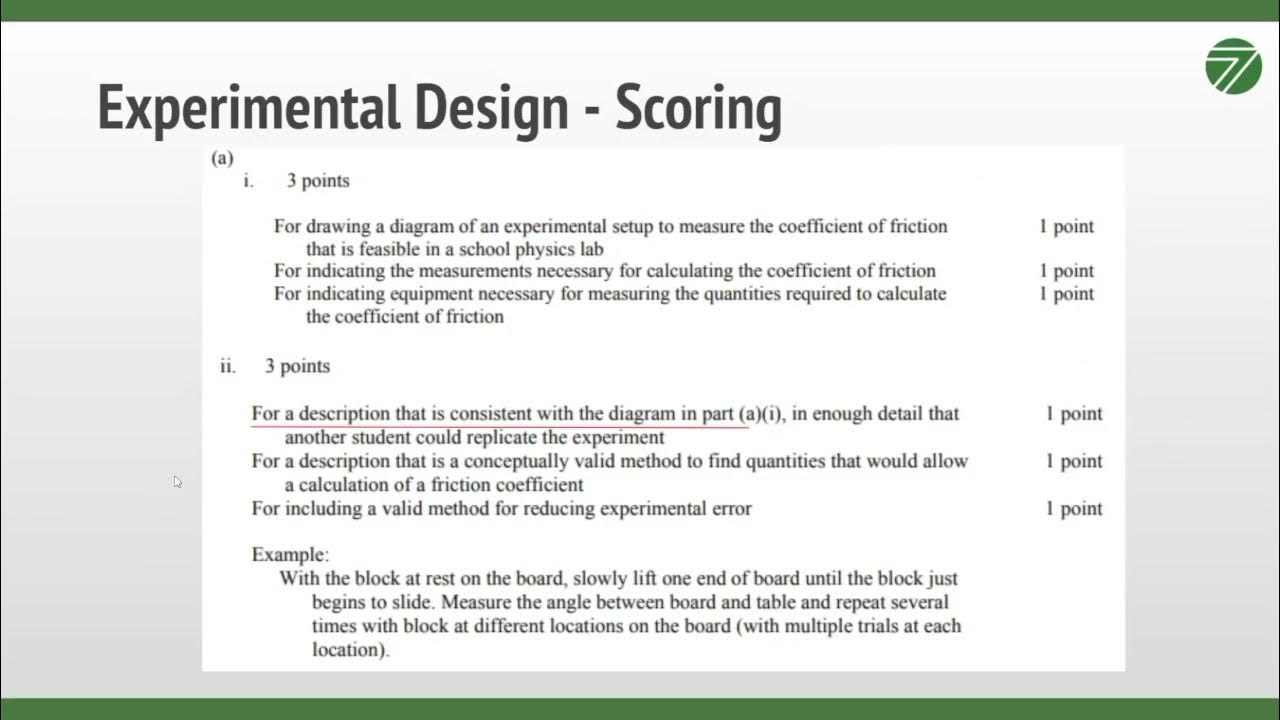The image appears to be a basic PowerPoint slide primarily used for explaining a scoring rubric for an experimental design assignment, likely intended for a college physics course. The slide is rectangular and horizontal, bordered by two dark green bands—one at the top and one at the bottom. In the top right-hand corner, there is a circular symbol containing an arrow-like shape made of two lines with green filling the middle. 

The headline, written in very large, bold-faced sans-serif type, reads "Experimental Design - Scoring." Below this, within a white block, the text begins with "A" in parentheses followed by "I" in parentheses and "three points." The first section details the points allocation: one point for drawing a feasible diagram of an experimental setup to measure the coefficient of friction in a school physics lab, one point for indicating the necessary measurements, and one point for listing the required equipment.

The next paragraph, indicated by "II" in parentheses, states that three points can be earned for a description consistent with the above diagram, detailed enough for another student to replicate the experiment. This includes providing a method for finding quantities to calculate the coefficient of friction and a valid method for reducing experimental error. The first sentence of this paragraph is underlined in red.

Following this, an example is provided: "With the block at rest on the board, slowly lift one end of the board until the block just begins to slide. Measure the angle between the board and table, and repeat several times with the block at different locations on the board, using multiple trials at each location." This illustrative example helps to clarify the instructions for students.